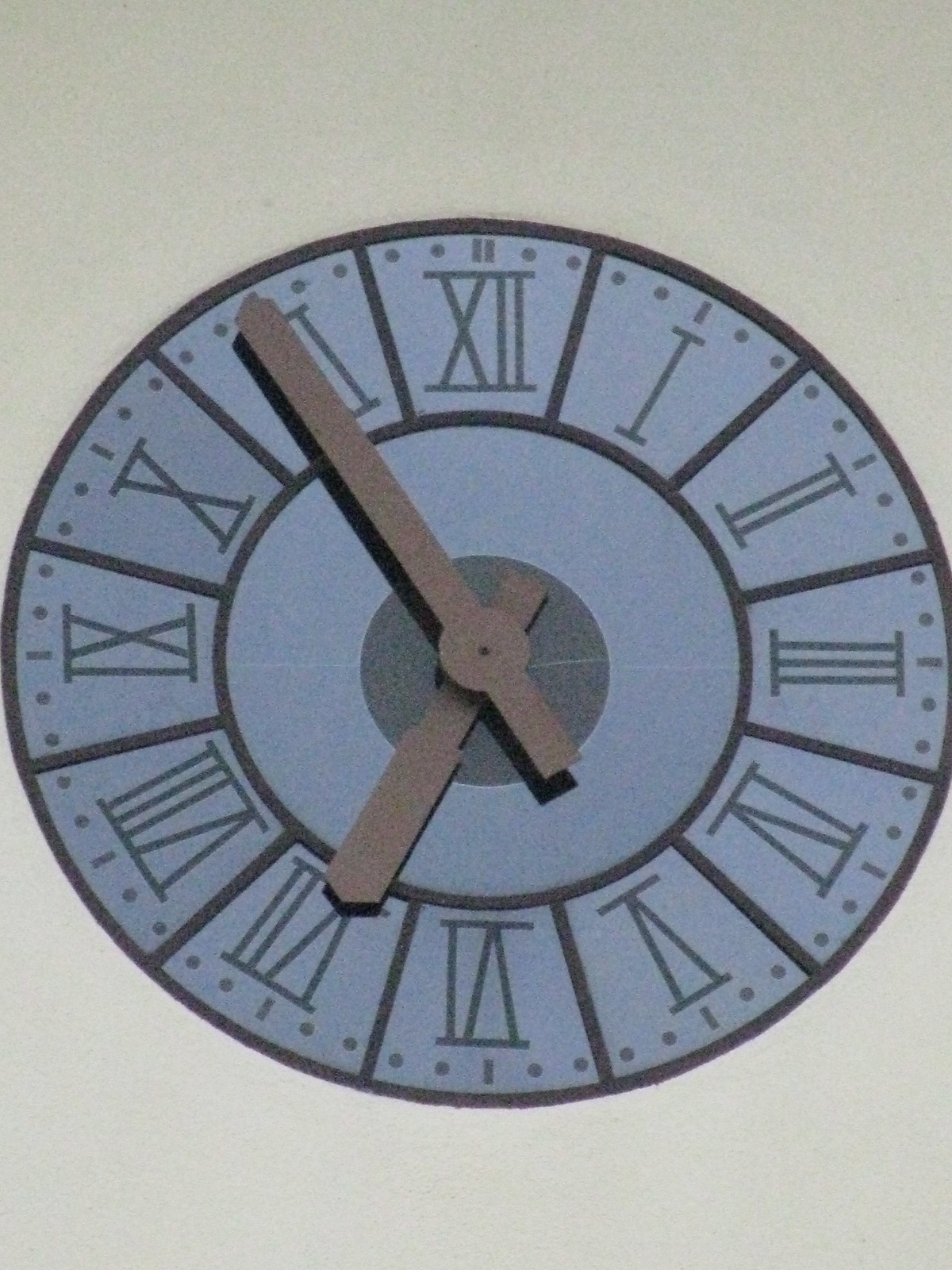The image showcases a painted clock, prominently displayed on a tan wall or building exterior. The clock itself features a blue circular background, with each Roman numeral framed in black, providing a striking contrast against the blue. The clock hands are brown and notably thicker than typical clock hands. At the center of the clock is a black circle, from which the hands emanate. The clock shows the time as 7:55, with the shorthand pointing at VII (7) and the long hand nearing XI (11).